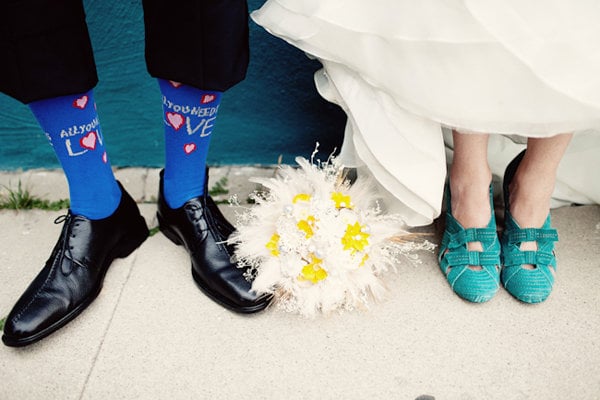This photorealistic image captures a unique and detailed view of a man and woman's feet, standing side by side on light gray sidewalk slabs. The man on the left wears polished black dress shoes paired with tall blue socks that feature white writing and pink and red hearts, forming the phrase "All you need is L♡VE." His black pants are pulled up, revealing a significant portion of the socks, suggesting a casual yet stylish look. The woman on the right, distinguished by her light skin tone, dons elegant teal high-heeled shoes. Her long white bridal gown is lifted slightly, showing part of her ankles and legs. Positioned between their feet is a white bouquet interspersed with bright yellow flowers, adding a touch of celebratory charm. The background features a blue-colored wall, hinting at an outdoor setting that might be near a pool, as indicated by some interpretations of the scene. This intriguing photograph, likely taken during a wedding, focuses closely on their feet and lower legs, emphasizing the blend of formal and sentimental elements.